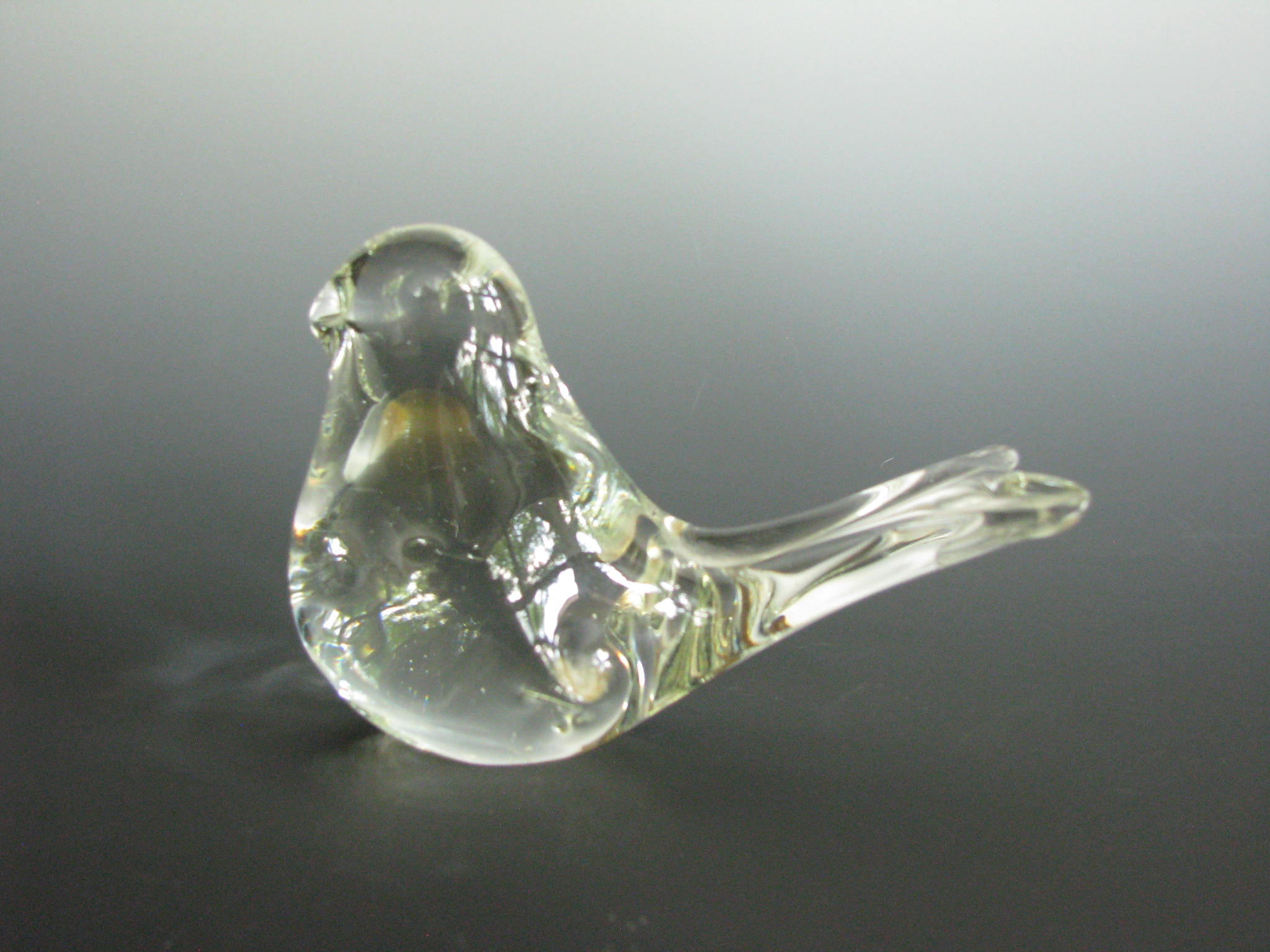The image showcases a simplistic yet captivating crystal bird set against a gradated gray to light gray background. The bird shape is rudimentary and basic, with clear glass that captures and reflects the surrounding environment, creating the illusion of embedded nature. Reflections of trees and plants enhance the visual complexity, appearing as if stems and leaves are within the bird's body. The figure, possibly a robin, has a discernible beak, elongated tail, and appears to be in a nesting posture, evoking a sense of familiarity despite its minimalist design. The craftsmanship hints at a novice creation, underscored by its unembellished form and transparent elegance.